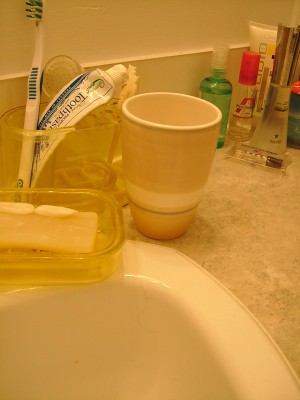This image captures a detailed view of a bathroom sink in a portrait orientation, lending a slightly narrow perspective to the scene. The sink itself is white and partially cut off, revealing approximately 30% of its bowl and a portion of the integrated white rim. Surrounding the sink is a firm, tan-colored surface exhibiting a subtle marbling effect, indicative of a solid countertop material.

The background of the photo is enveloped in a yellowish hue, possibly due to the room's lighting or a camera effect. A tan border runs along the white wall above the sink, adding a touch of contrast.

On the countertop, various items are neatly arranged. On the left side, there is a yellow, oval-shaped container holding a bar of soap. Above it, a transparent yellow container housing a toothbrush and toothpaste is positioned. Next to this, a cup likely used for rinsing is placed casually.

Further to the right, in the upper corner of the image, there are several bottles. The lineup includes a clear green bottle with liquid, a transparent bottle that appears to be cologne, and another clear bottle topped with a red cap, possibly containing another type of liquid product. The meticulous arrangement of these everyday items provides a snapshot into the practical functionality and daily routines of the bathroom space.